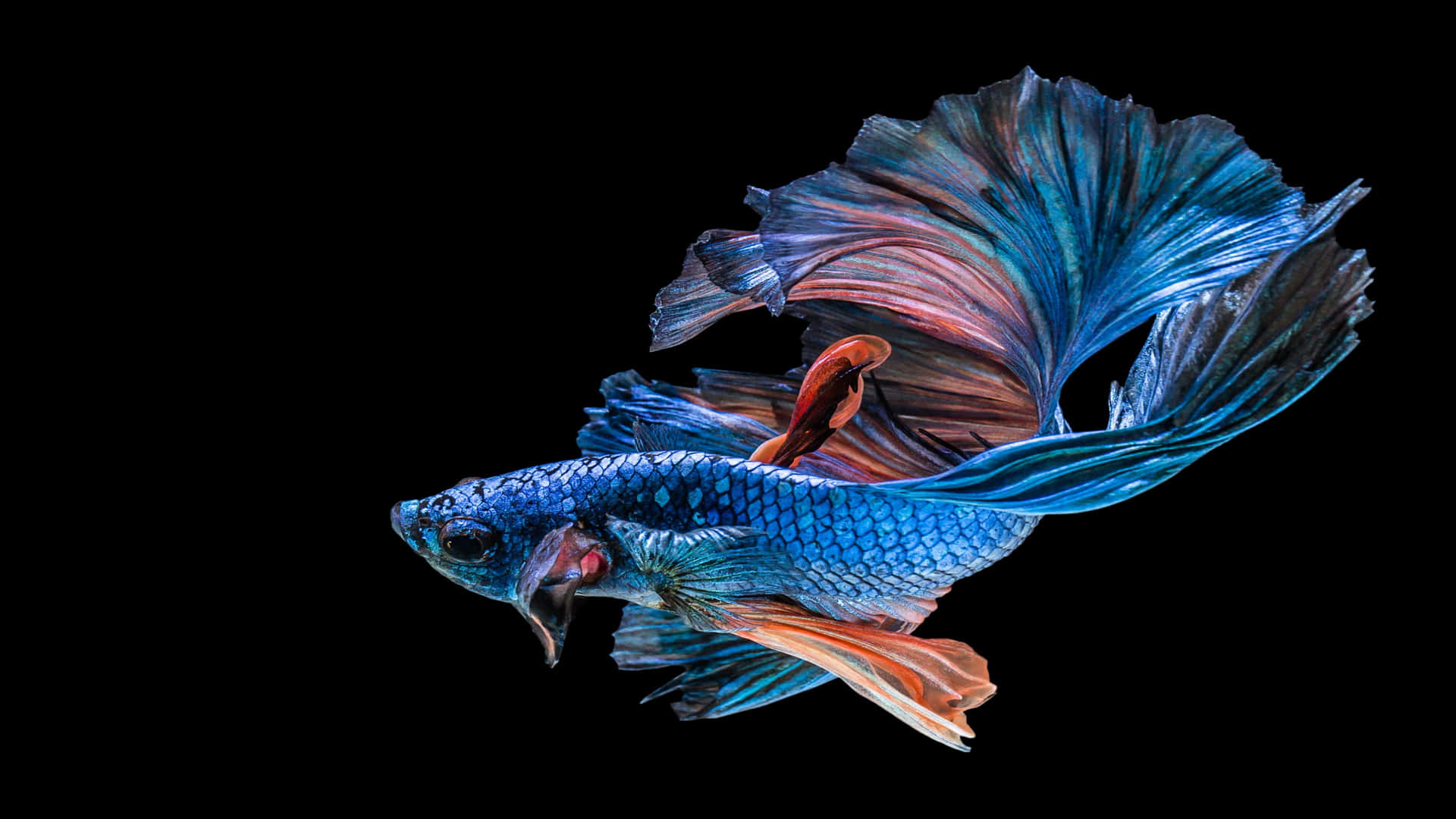This image showcases a digital painting of a strikingly beautiful beta fish set against a solid black background. Central to the composition, the fish captivates with its elongated fins and tail, which fan out elegantly, occupying more space than its body. Predominantly blue, the fish features rich, dark blue tones around its gills and head, which is facing left and adorned with a prominent dark eye. Accentuating its vibrant blue are striking orange highlights, particularly on the fins and tail, which display additional hues of purple, turquoise, green, and even pink. The artistic rendering gives the fish a dynamic, almost ethereal appearance, with the delicate interplay of colors adding depth and visual interest to the otherwise minimalist scene.